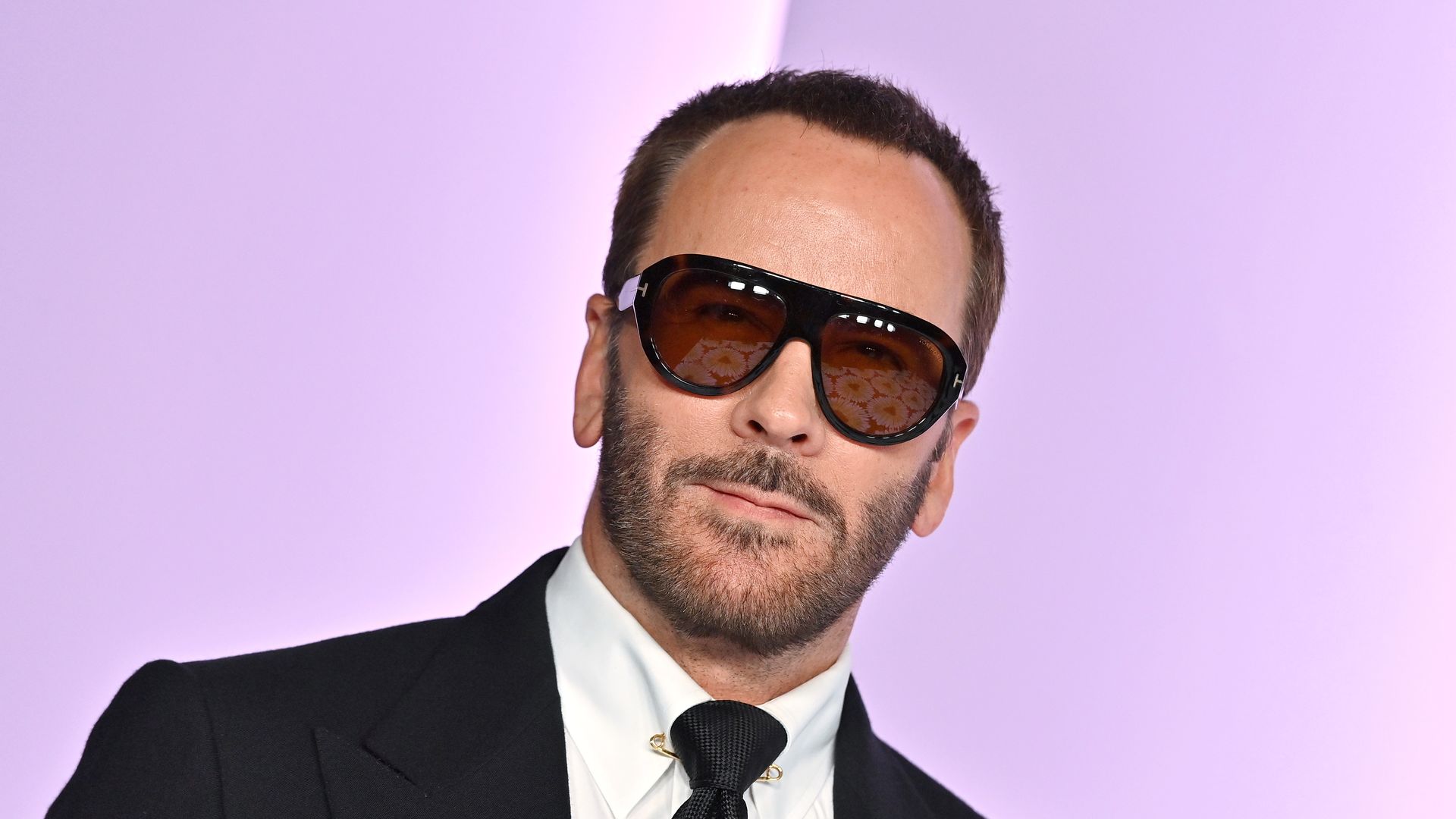This photograph features a well-to-do man standing against a muted lavender background that has a faint two-toned quality. He has neatly cropped short hair with a receding hairline and a tanned complexion. His facial hair is styled in a Van Dyke with a short beard and mustache. His attire consists of a sharp black suit, a white shirt, and a black tie, and there is a gold safety pin fastened behind the tie. The man sports a pair of large, thick-framed sunglasses with muted amber lenses that reveal his dark eyes behind them. Reflections in the lenses give off a glare that might include an image of pies from a bakery and some patterned cloth. He is leaning slightly to his left and has a hint of a smile on his face, which together with his overall appearance, projects confidence and affluence.